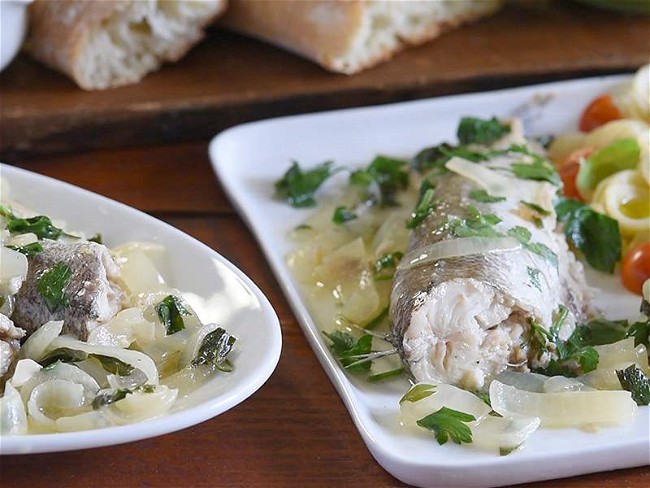In this photograph, we see a rustic and inviting restaurant setting, showcasing two white plates of a meticulously prepared fish dish on a dark wooden table. The foremost plate on the right is square with rounded corners, featuring a whole poached or boiled fish with its skin intact, garnished with cooked onions and a scattering of vibrant green herbs, possibly parsley or cilantro. Adjacent to this, within half an inch, is a partially visible oval plate containing the same dish, echoing the delightful arrangement of fish, onions, and greens. The background reveals a small shelf holding rustic loaves of fresh, crusty bread, already cut and partially broken open, adding to the homely and hearty atmosphere of the scene. The overall presentation suggests a nutritious and flavorful meal, rich in visual and culinary appeal.